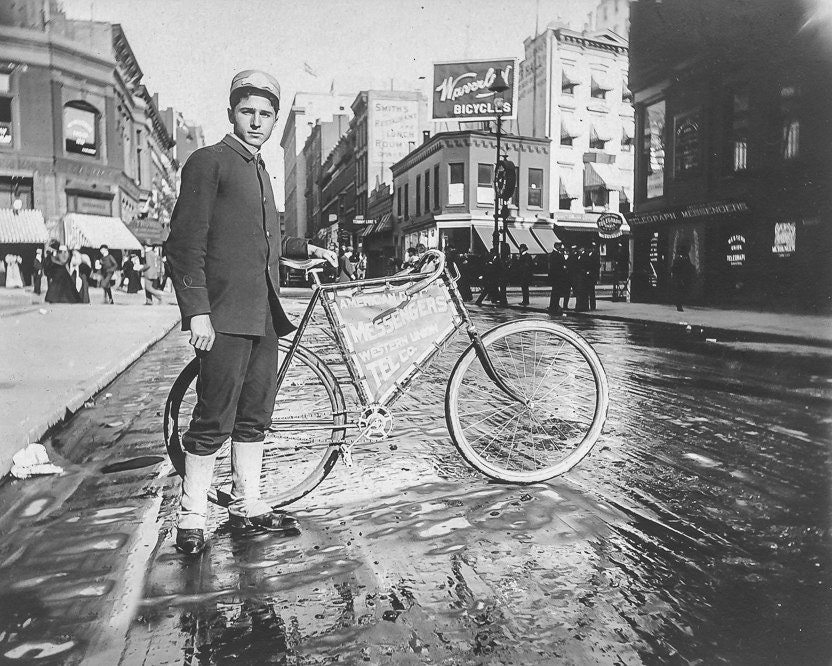In this vintage black-and-white photograph from the early 1900s, a middle-aged white man stands proudly in front of an old bicycle with distinctive white-walled tires and small, white spokes. The bicycle, featuring very large wheels, a high seat, and a low handle, hints at its age and possibly the man's role as a newspaper delivery boy or messenger, as an advertisement on the bike suggests. The man is well-dressed in dark clothing, including knickers that reach just below his knees, long white socks, and black shoes. He also wears a dark jacket and a light-colored messenger hat with an emblem on the front and a small bill. He is looking directly at the camera, his expression serious and focused.

The setting is a wet, shiny road, which could be due to recent rain or possibly oil covering the dark surface. Flanking the road are dry, gray sidewalks. In the background, we see an old-style cityscape with various buildings, one prominently reading "Woodrun Bicycles," suggesting a connection to the bicycle company. On either side of the central bicycle store are more stores with well-dressed men standing in front of them, highlighting the early 20th-century atmosphere. The photograph captures a distinct moment in time, reflecting both the man's occupation and the era's urban environment.